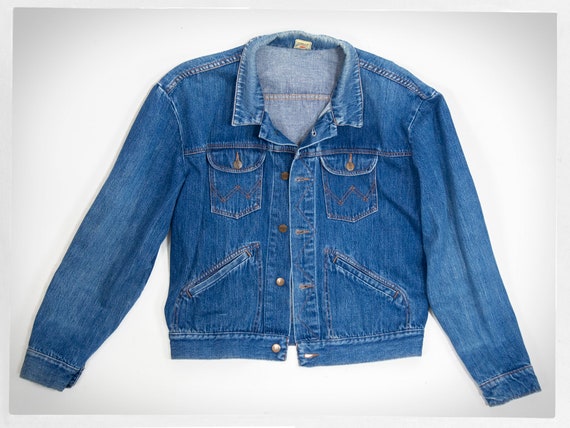This image features an older, vintage blue denim jacket, likely from the seventies, mounted in a light white frame against a whitish-gray background. The jacket appears to be small, possibly designed for a woman, and is displayed closed but not fastened, with the collar open. There is a small tag on the top of the back collar. The jacket includes four pockets: two chest pockets with gold buttons for closure and two lower hand pockets angled for easy access, also adorned with goldish-silver buttons. The front of the jacket sports five buttons in total, with one specifically for the collar. The detailed stitching and vintage design elements further emphasize its retro appeal.